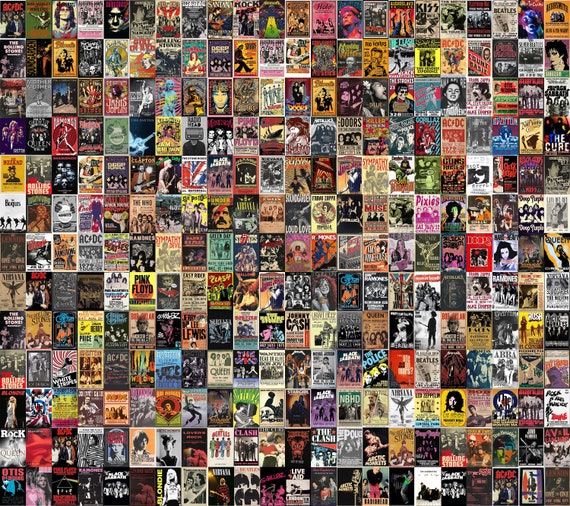This is a highly detailed and colorful illustration arranged in a square format, featuring a collage of what appear to be hundreds of tiny album covers or posters, all related to rock music. The grid-like arrangement includes 13 rows and 21 columns, displaying a vibrant mosaic of diverse artwork and text. Prominent among the recognizably featured artists and bands are The Doors, Nirvana, The Pixies, The Police, Queen, Pink Floyd, Jimi Hendrix, and Miles Davis. Each small square within the collage is distinct, contributing to a busy and dynamic visual experience teeming with colors and intricate details. This image resonates with the essence of rock music history through its rich array of miniature posters.